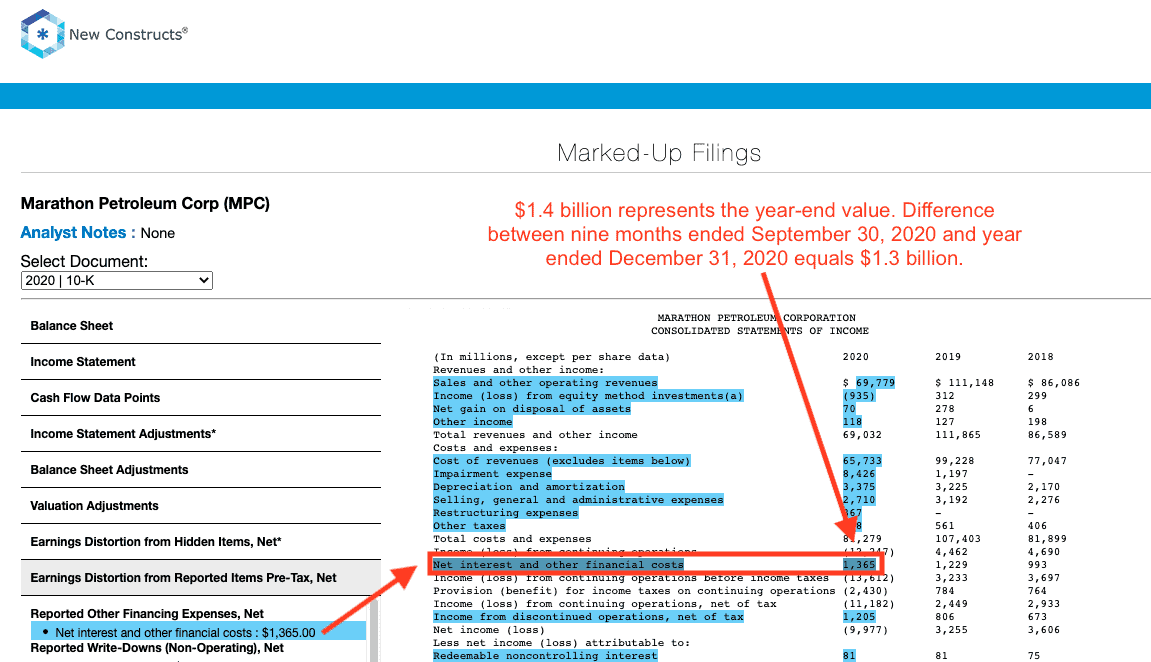The image features a highly detailed financial document with a blue header and various highlighted sections. In the background, new constructs are visible. The red text indicating "1.4 billion" highlights the year-end value difference between the nine months ending on September 30th, 2020, and the year ending on December 31st, 2020, which equals 1.3 billion. A red arrow points to the numeric value 1,365, which is prominently highlighted in blue. To the left of this figure, the phrase "Net Interest and Other Financial Costs" is also highlighted in blue. Another arrow indicates this section, originating from the line specifying "Net Interest and Other Financial Costs: $1,365." Additionally, the text notes "Marathon Petroleum Corp (MPC)" with analyst notes in blue stating "None." The document header reads "Select Document 2020" and includes a dividing line. Below this, several line items are listed: "10K Balance Sheet," "Income Statement," "Cash Flow Data Points," "Income Statement Adjustments" with an asterisk, "Balance Sheet Adjustments," "Valuation Adjustments," and "Earnings Distortion from Hidden Items Net" also marked with an asterisk.